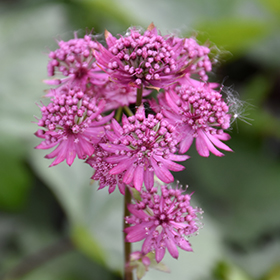This is a detailed outdoor close-up photograph of a pink to purple wildflower in full bloom. The central focus of the image is the sharp, vividly captured flowers, each showing a burst of approximately 15 small, pointed petals arranged in a circle. Emerging from a single green stem, there are about six to eight open flowers, each with a prominent cluster of 20 to 30 pestle-pointed bulbules at their centers. The thin, elongated oval leaves and buds associated with these flowers also appear prominently. The background is a beautifully blurred green, typical of bokeh effects, creating a soft contrast with subtle hints of lighter white-green areas, likely from other distant foliage. The overall appearance of the scene suggests a natural, wild setting rather than a cultivated garden.